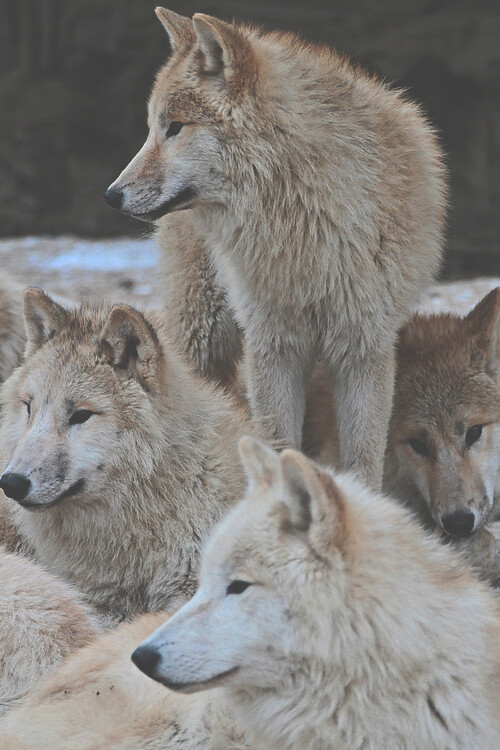This is a professional, vertical photograph of a pack of six Arctic wolves, possibly hybrids with a coyote due to their smaller stature and distinct features. The wolves are predominantly light brown with a reddish tint on the tips of their fur, underneath which lies a white and gray coat. Some wolves have additional black or white markings on their elongated snouts. The pack is situated outdoors, with a background that suggests a snow-covered, blurred forest. A lone wolf stands at the center of the frame, its tan fur speckled with darker brown, dark brown ears, and a black nose. This wolf looks to the right, while three others lie close by, with two also gazing right and one looking directly at the camera. The remaining wolves' bodies are partially visible but obscured. All wolves have bushy coats, closed mouths, and the same coloration pattern, giving the photograph a mix of detailed clarity and a natural, almost painting-like quality despite the indistinct background.